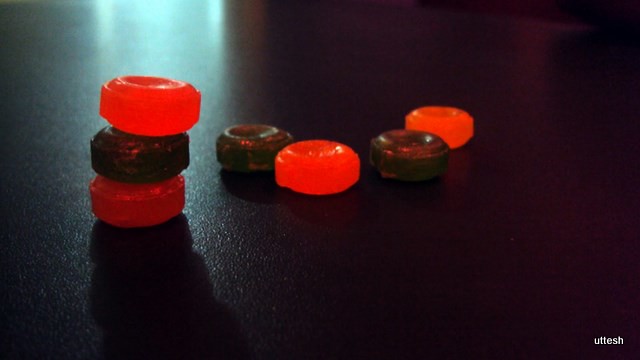The image features a very dark photograph with a black table surface illuminated softly towards the upper left-hand corner. Prominently displayed are hard candies, reminiscent of lifesavers, in vibrant red and black colors. The composition prominently shows three circular candies stacked one on top of the other towards the left side, with a red candy at the top, followed by a black one, and another red one at the bottom, slightly tilted to the right. In the background, additional candies are scattered flat on the table. This arrangement includes two red pieces and two dark candies that appear black but exhibit a subtle greenish tint under the lighting, adding a nuanced depth to their color. The candies are shiny but captured in a muted color palette. There is typewriting in white at the bottom right of the image, spelling "Altesch." The overall scene is one of a starkly lit, high-contrast display, enhanced by the strategic light reflections that cast a subtle glow on the table and candies.